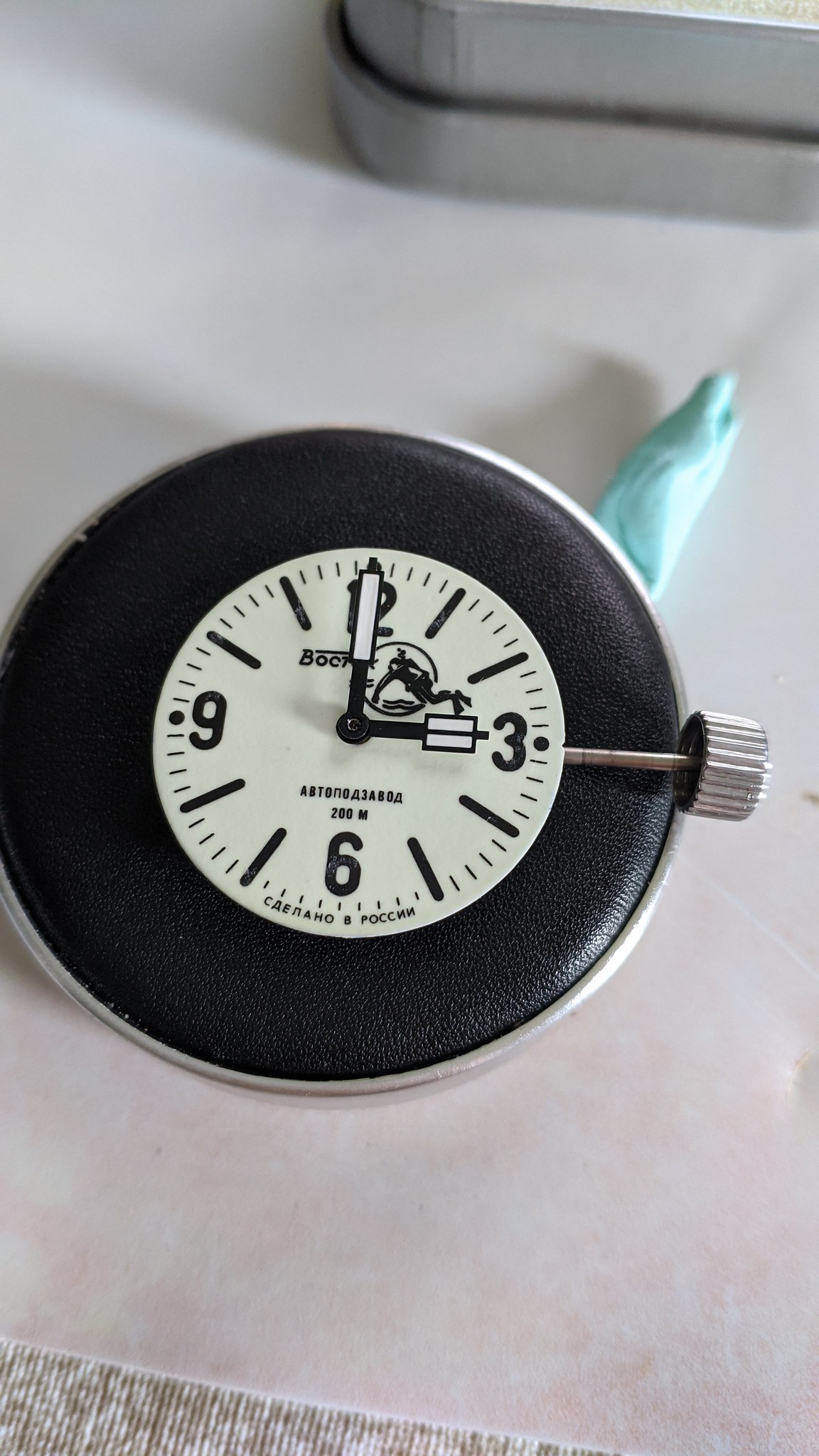The image features an unusual and intricate pocket watch centered prominently. The watch is circular with a black, textured leather outer ring and a white clock face. It has a visible winding stem situated on the right side, intriguingly lying atop the clock face. The face displays only the numbers 12, 3, 6, and 9, with black markings against the white background, while slender black and white minute and hour hands point to three o'clock. 

The backdrop consists of layered surfaces, including a beige and white textured material, potentially resembling vegetable paper, overlain by a light pink and white surface. The metallic, silver outer edge of the watch contrasts with the black leather, and there’s a peculiar detail of light green material at the top, perhaps indicating an attempt to fix the watch. The watch face features large lines for the main hour markers and smaller ones for the minutes.

Adding to its peculiarity, the watch brand name, somewhat illegible, might read "BOC ...", paired with the image of a diver in a wetsuit. Below this, there are cryptic letters and numbers, "A, B, T, 0, N, 0," alongside more characters which appear to be Cyrillic, hinting at a Russian origin with markings like “P, O, C, C, backwards N, backwards N," possibly signifying Russia. The depth rating “200M” further adorns the watch face, suggesting it is water-resistant up to 200 meters. All these layers of details make the watch uniquely complex and visually captivating.